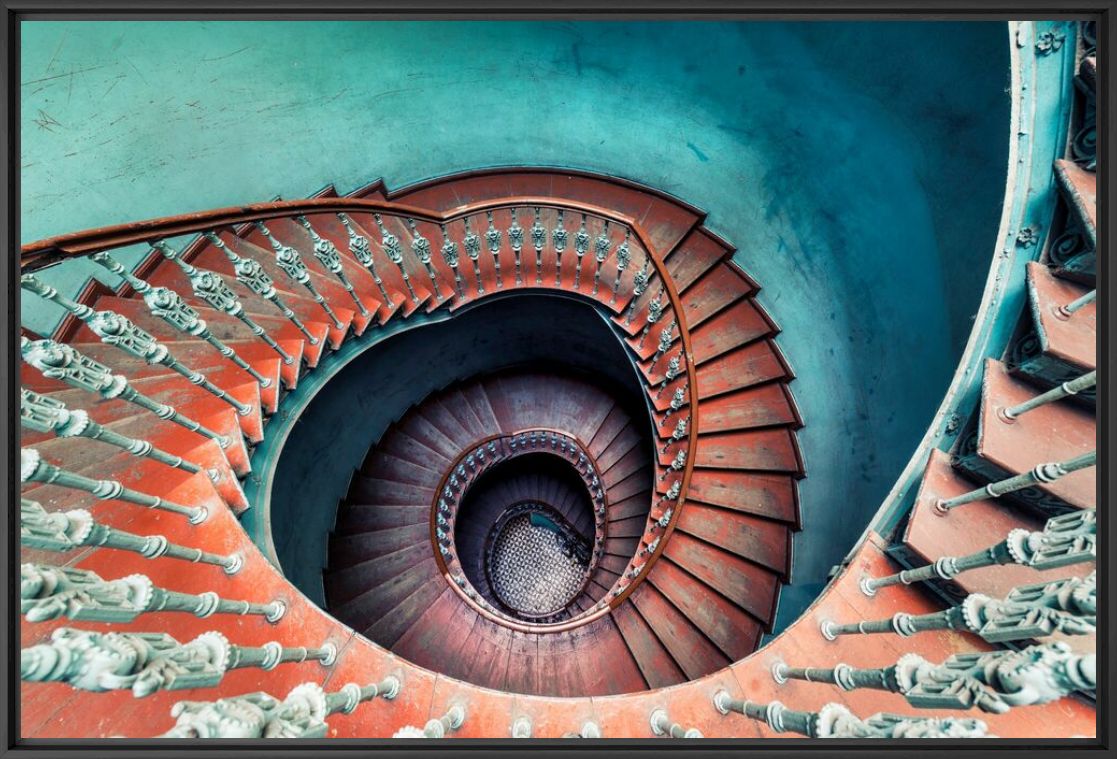This image features an aerial view of a grand, spiral staircase that twists around in a modern contemporary style. The staircase has multiple flights, spiraling downwards, creating a captivating visual effect. The steps appear to be an orange mahogany color, with visible discolouration that reveals a greyish tone in the center, likely from years of foot traffic. The railing is a dark, reddish-brown with white accents, and the spindles are a silvery color, potentially designed to resemble human figures. The surrounding walls are a striking turquoise blue, akin to the color of the sea. At the bottom of the staircase, the flooring appears to have a patterned design, possibly a black and white checker pattern. The overall ambiance of the staircase, though perhaps aged, is rendered with a modern aesthetic, possibly enhanced by a photographic filter. The image may be set inside an architectural structure such as a lighthouse, given the spiraling design and towering height.